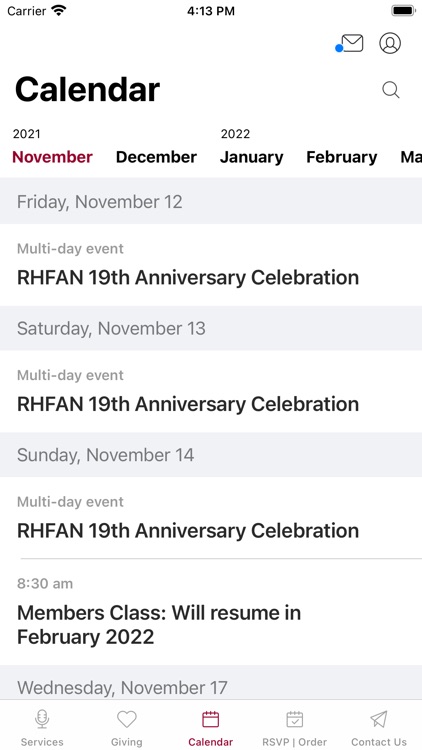This is a detailed screenshot from a cell phone, displaying a calendar application. The background is white with light gray horizontal bars. 

At the very top, the left corner shows the text "carrier" and the Wi-Fi symbol. The center of the top bar displays the time as 4:13 p.m., and the top right corner features a full battery icon. Just below this bar, on the right side, there are envelope and profile icons.

The first line of the main content is dominated by the bold, large, left-justified word "Calendar." Directly under this, there are month indicators: "2021 November December" and "2022 January February March," with "November" selected.

Below the month selectors is a light gray box displaying "Friday, November 12," followed by the event "Multi-day event RHFAN 19th anniversary celebration." The same structure continues for "Saturday, November 13" and "Sunday, November 14," each accompanied by the same multi-day event.

A thin gray line separates these entries from a second entry for "8:30 a.m. Members class will resume in February 2022." The next gray box at the bottom of the screen notes "Wednesday, November 17."

At the bottom of the screen, there are several icons with corresponding labels: a chair icon labeled "Services," a heart labeled "Giving," a highlighted calendar indicating the current selection "Calendar," an RSVP/order option, and a paper plane icon labeled "Contact Us."